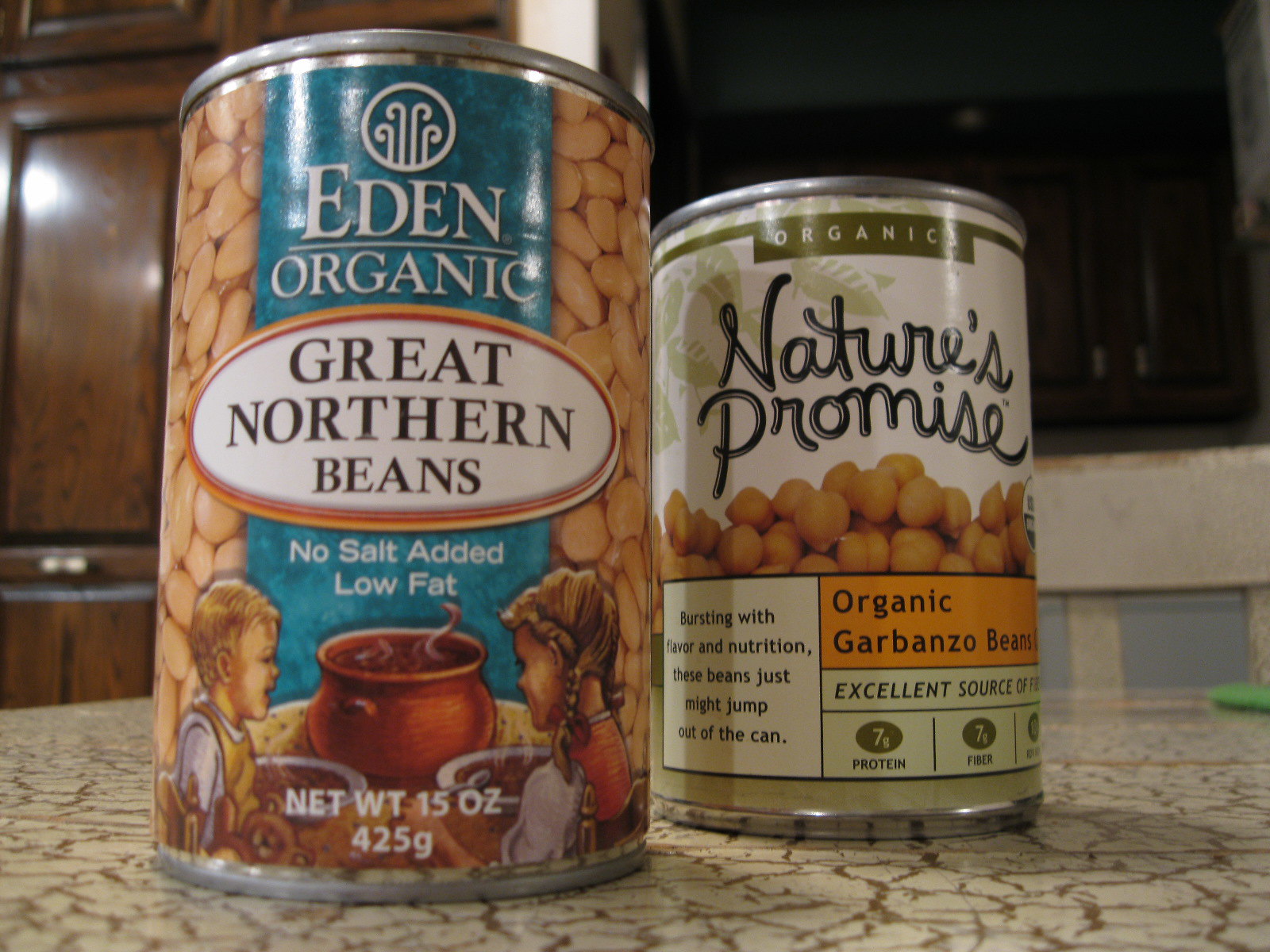The image features two cans of beans placed on a white countertop with brown lines. The can on the left, positioned slightly closer to the camera, features a label that reads "Eden Organic." Above the text is a white circle emblem with a stylized graphic, resembling a person blowing upwards. The main text in the center of the label says "Great Northern Beans" in black, set within a white oval bordered by an orange rim. Below, the label notes "no salt added" and "low-fat." An illustration decorates the lower section, depicting a boy on the left and a girl on the right, both holding bowls, with a brown cooking pot positioned between them. A blue strip serves as the background for this illustration, flanked by images of beans.

The can on the right is set against a green and white background adorned with leaf motifs. The label displays "Nature's Promise" along with "organic garbanzo beans." Although partially obscured, the text mentions the beans being an "excellent source of" something, and emphasizes their vibrant flavor and nutrition with the tagline, "bursting with flavor and nutrition these beans just might jump out of the can."

The cans rest on a white countertop with brown lines. In the background, the right side features a black object that appears to be a television, accompanied by a plant. On the left side of the image, brown kitchen cabinets are visible.